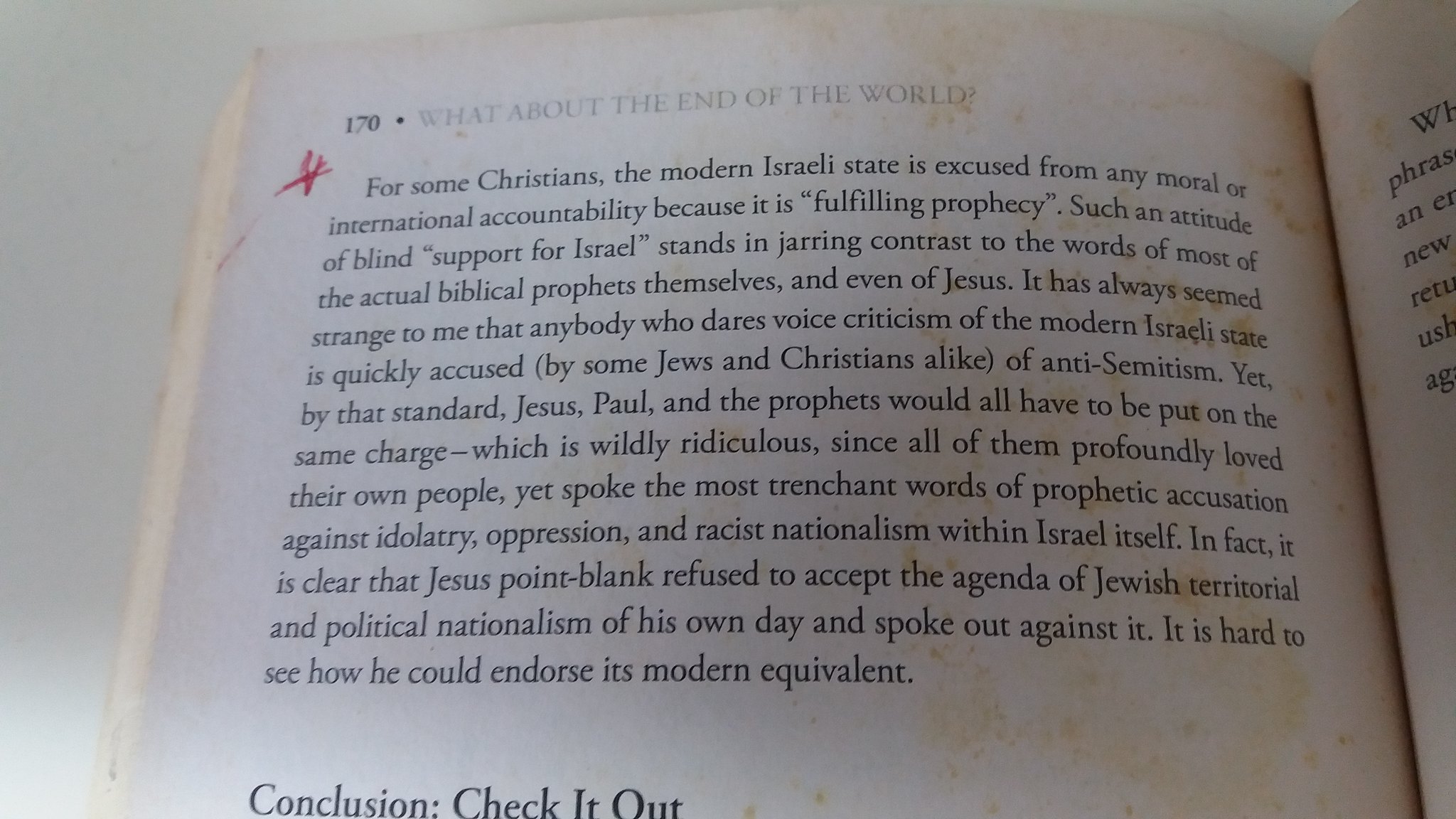The image shows an open page of a book, specifically page 170, marked by a red pin below the page number. The chapter is titled "What About the End of the World?" The text discusses the perspective of some Christians who excuse the modern Israeli state from any moral or international accountability because they believe it is "fulfilling prophecy." The author contrasts this "blind support for Israel" with the words of many biblical prophets and Jesus himself, who often criticized idolatry, oppression, and racist nationalism within Israel. The text argues that labeling criticism of the modern Israeli state as antisemitism is illogical, as it would similarly label Jesus, Paul, and the prophets, who loved their people yet spoke against such issues. It emphasizes that Jesus explicitly rejected Jewish territorial and political nationalism in his time, making it difficult to believe he would endorse its modern counterpart. At the bottom, in bold letters, is the word "Conclusion" followed by the phrase "check it out."